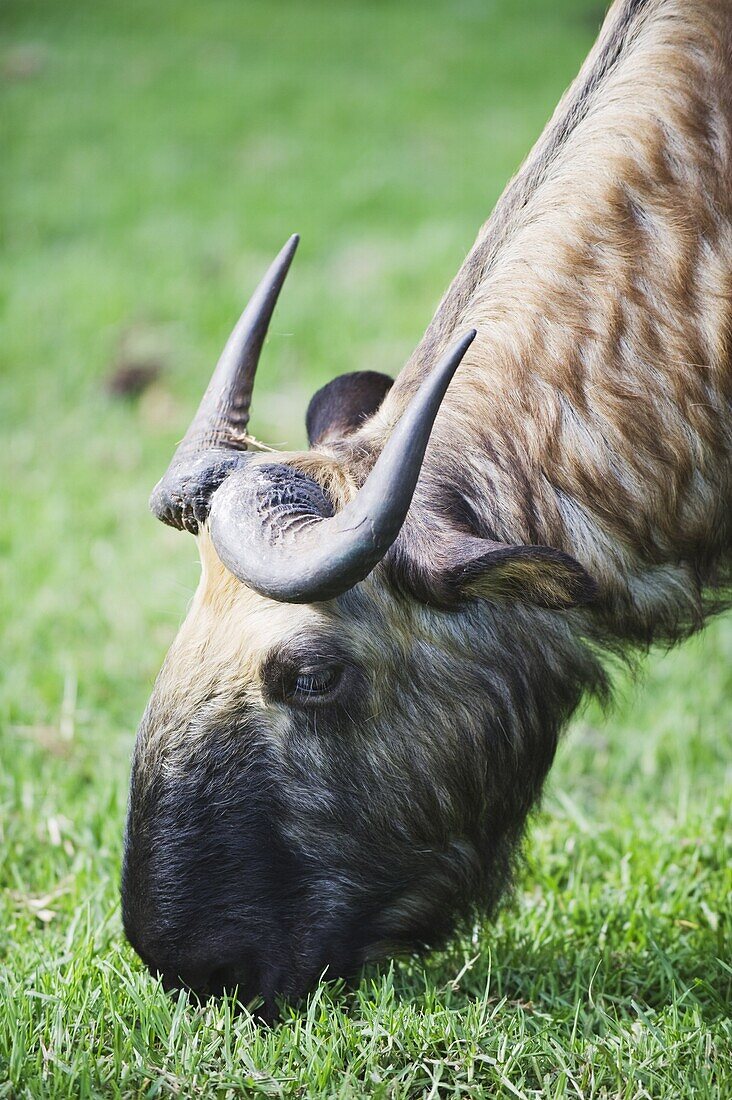In this vertical rectangular image, a cute animal—possibly a cow or bull—is depicted in a close-up shot as it eats grass. The animal's head and neck dominate the frame, with its neck starting in the upper right corner and extending down to the lower left where it reaches for the grass. Only one eye is visible in this profile view, while the rest of its face, including the nose and mouth, is hidden in the grass. The creature has two sharp, black horns positioned symmetrically on its head, with a single visible ear located just behind the nearest horn. Its fur features alternating light brown and white patches, creating a fluffy texture. A darker stripe runs down the back of its neck, contrasting with the lighter colors. The scene is set in daylight, and the absence of any text directs full attention to the animal and its serene activity.